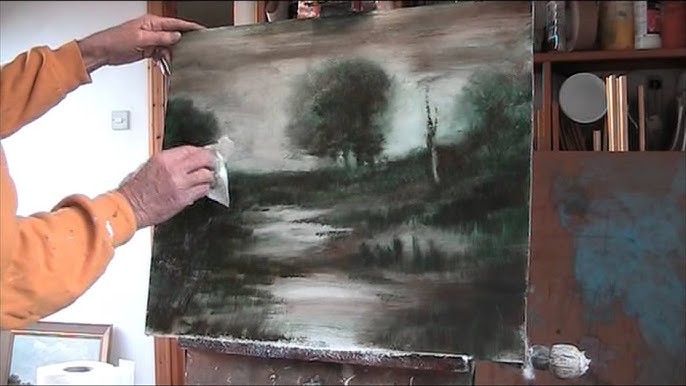In this image, an older man, dressed in a peach or light orange shirt with paint-stained hands, is delicately wiping a canvas painting with a paper towel or tissue. He is using his right hand to clean or blend parts of the painting, while his left hand steadies the artwork. The painting itself portrays a gloomy forest scene with dark green and gray hues, featuring two trees, a small lake to the left, and a sky that appears brown, white, and gray. The painting leans against a surface, likely in a studio or labor room, with a brown shelf in the background holding various artist's utensils. Additional supplies, including a roll of toilet paper and possibly another small painting, are visible at the bottom left of the scene.